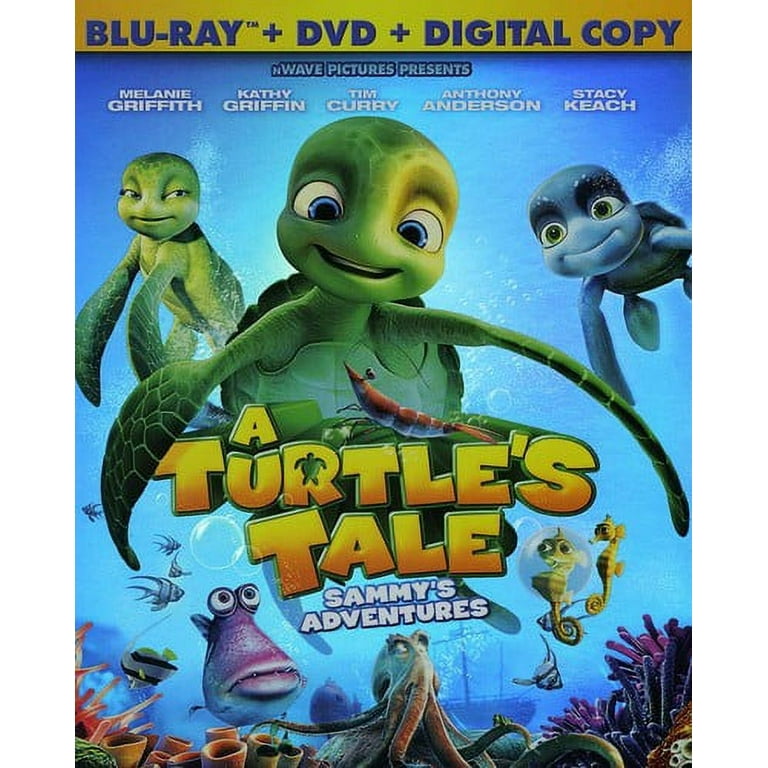The Blu-ray cover features a vibrant ocean background showcasing an array of underwater life. The top portion is deep blue, bordered by a bright yellow bar containing blue text that states "Blu-ray + DVD + Digital Copy." Below this, "N-Wave Pictures Presents" is prominently displayed, followed by the names of the voice actors: Melanie Griffith, Kathy Griffin, Tim Curry, Anthony Anderson, and Stacey Keach, all in white text that stretches across the cover.

Dominating the middle section, three turtles with large, expressive cartoon eyes and human-like mouths gaze towards the viewer. Among them, two are green and one is blue. The movie's title, "A Turtle's Tail," appears in a distinctive yellow-to-orange gradient font with a small turtle icon in the letter 'R.' Underneath, "Sammy's Adventures" is written in white text with a blue outline.

The lower section is abundant with colorful sea creatures, including a big pink fish with a large mouth and quirky eyes, yellow seahorses peering at the title, an octopus, angelfish, coral, and a grouper. Additionally, a shrimp is seen perched on the title, adding to the lively, whimsical underwater scene.